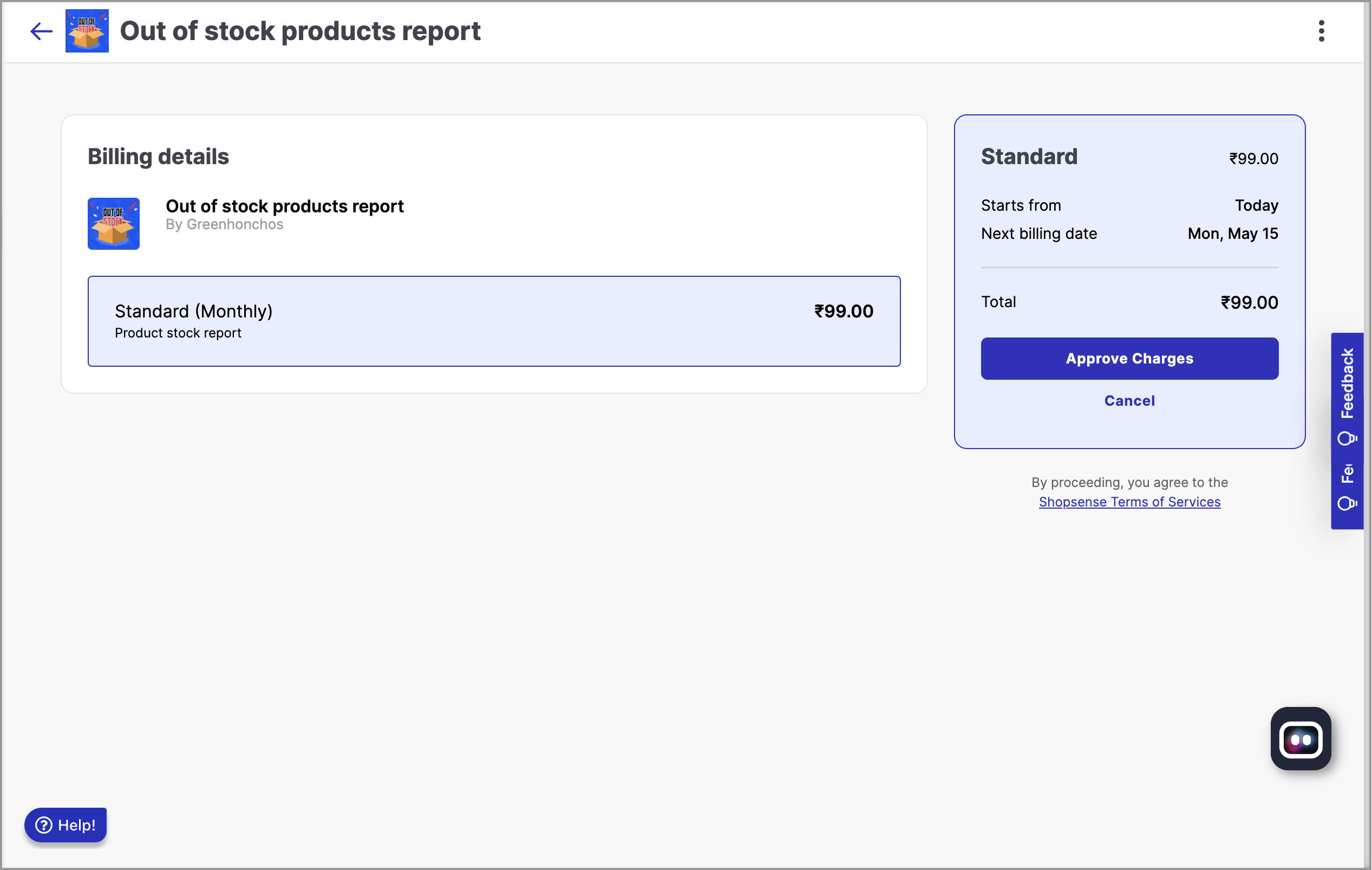This is a screenshot of a webpage displaying an "Out of Stock Products Report." In the upper-left corner, there is a left-pointing arrow, seemingly a back navigation button. Next to it, there is a blue icon featuring an open cardboard box. To the right, the heading reads "Out of Stock Products Report." 

In the upper-right corner, three vertical dots indicate a dropdown menu. Below the main header, in a white rectangle, it says "Billing Details, Out of Stock Products Report by Green Honchos." Below, there's another blue icon of an open cardboard box labelled "Standard," with the note "(Monthly Product Stock Report)" priced at $99.

To the right of this section, there is a blue button with the text "Standard" in black letters, and below it, "$99." The text further specifies "Starts from today, next billing date Monday, May 15th, total $99 approved charges." There's also a blue button with white text, and just below it, the word "Cancel" appears.

At the bottom of the section, there's a disclaimer stating: "By Proceeding You Agree to the ShopSense Terms of Services," with "ShopSense Terms of Services" being a clickable blue hyperlink. In the bottom-left corner, there's a blue "Help" button, and in the bottom-right corner, there's another small, unspecified box.